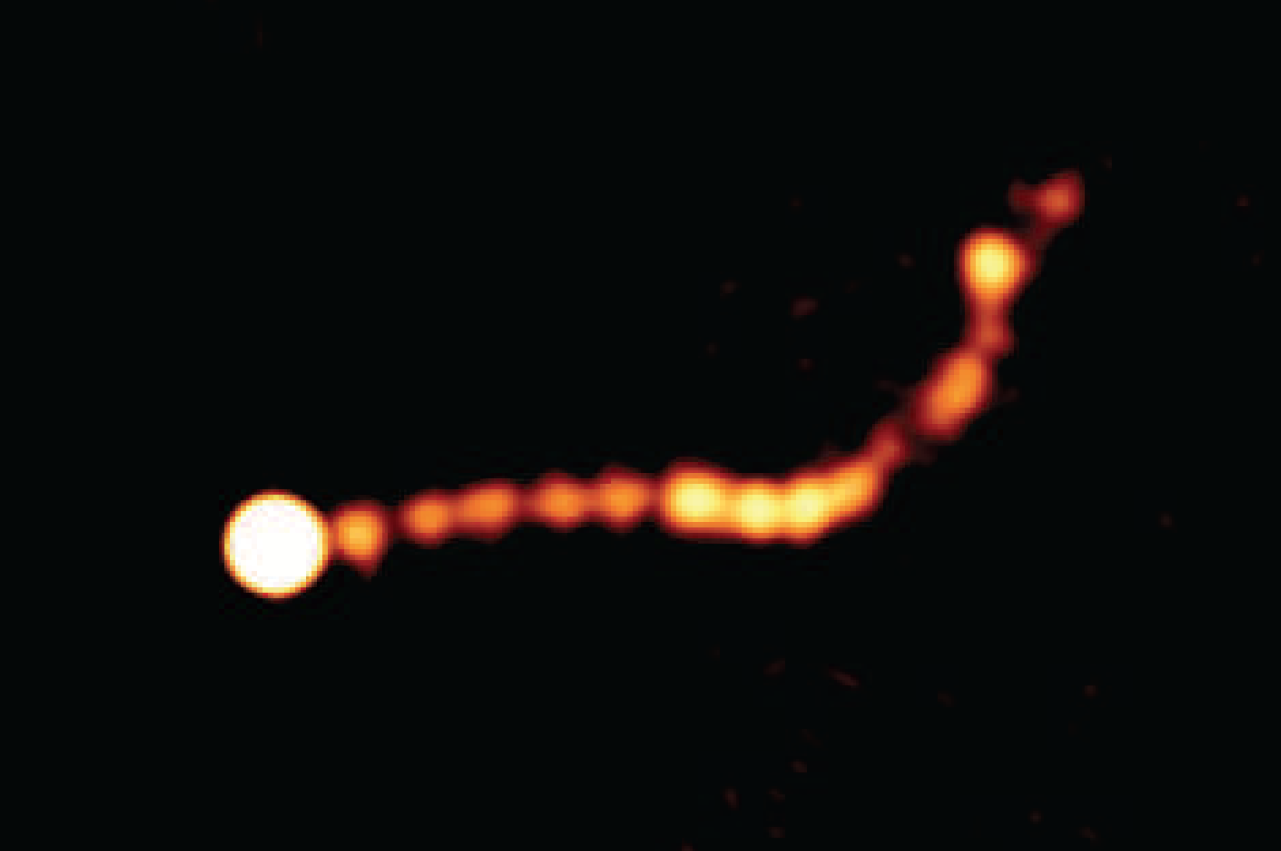In a predominantly black and rectangular image, the photograph captures a visually striking scene dominated by a fiery phenomenon. At the center, positioned slightly towards the bottom left-hand corner, is a glowing white circle with an intense orange aura, resembling a brilliant fireball. This central sphere appears to be the focal point of the image, accentuated by a distinctive tail of orange, red, and yellow hues that curves upward, giving the impression of a trailing streak through the dark sky. Along this trail, there is a sequence of smaller luminous dots; the initial five are orange and dimmer, followed by four slightly larger and whiter, more intense dots, culminating in a few more variably bright dots. These details create the illusion of a chain of light digitized in slow motion, amplifying the mystique of the image and its fiery subject. The photograph, although dark and somewhat pixelated, vividly captures the mesmerizing path of what suggests a fireball or a slowed-motion streak of light amidst a night sky.